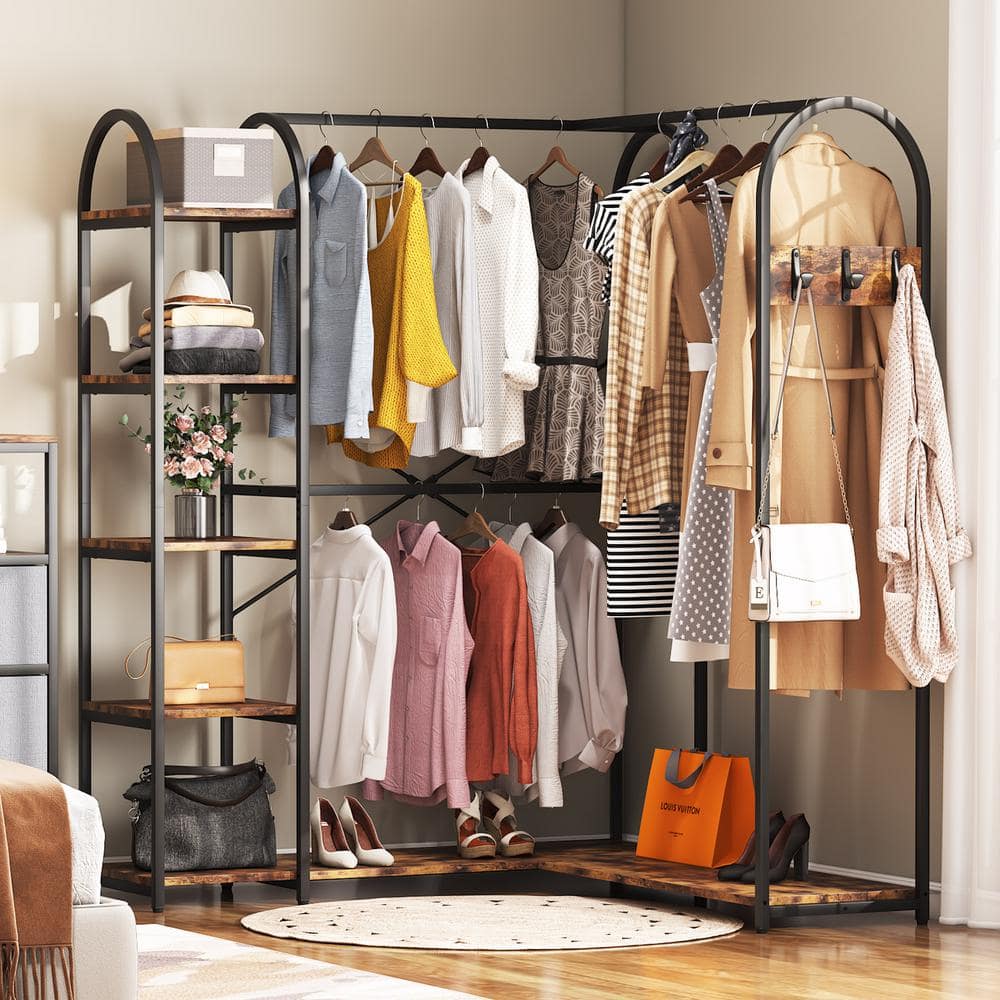In the corner of a room with light gray walls and light brown hardwood flooring, there is an L-shaped portable closet apparatus made of black metal bars with wooden shelves. This corner clothes organizer fits perfectly and features a combination of hanging spaces, shelves, and hooks. The left section has two levels for hanging various women's clothes, including dresses and casual outfits, while the right section has space for jackets and a long trench coat. The top of the organizer has an arched metal structure with a connecting bar, providing additional hanging space. 

There are five wooden shelves connected to the structure, featuring different items on each shelf: the top shelf holds a shoe box, the second shelf has folded clothes with a hat on top, the third shelf displays a silver vase with light pink flowers, the fourth shelf contains a light brown handbag, and the bottom shelf accommodates a large black shoulder bag. At the base of the unit, there is an L-shaped wooden shelf for placing shoes or purses, with high-heeled shoes prominently displayed. On the side hooks, a purse and a sweater are hung. This detailed and functional closet system is versatile enough for both home use and retail display.